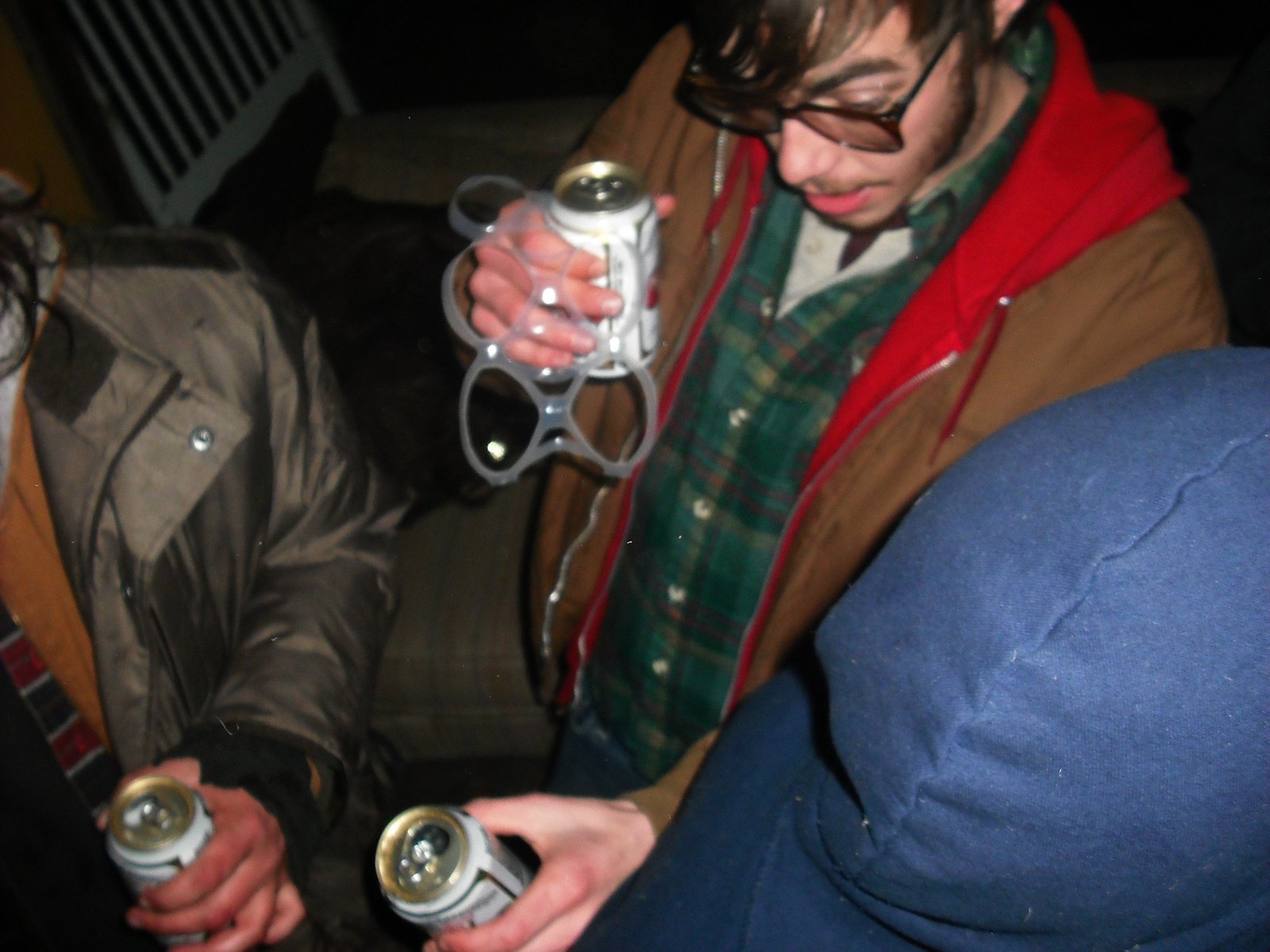In this nighttime outdoor scene, a group of men is gathered for an informal get-together, each holding cans of beer. The focal point is a man with dark hair, thick black eyebrows, a light dusting of beard stubble, and black-rimmed glasses. He sports a green plaid button-up shirt beneath a brown jacket, which appears to have a red lining. In one hand, he clutches a white and gold beer can still attached to the plastic from the pack, while his other hand holds an open can of the same brand. To his left, part of another man is visible, identifiable by his gray jacket and a glimpse of an orange shirt beneath it, also holding a beer can. In the upper left corner of the image, another individual appears, facing downward; he has dark hair and black glasses, wearing a similarly attired green plaid shirt under a brown jacket. On the right side, a man in a blue hooded sweatshirt is present, though only his back is visible. The group is evidently dressed warmly for the outdoor night, emphasizing the casual and convivial atmosphere of their gathering.